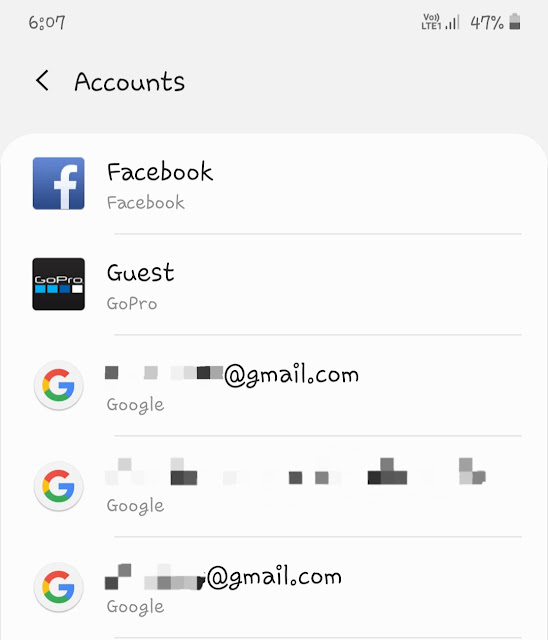The image appears to be a stylized, hand-drawn rendering of a smartphone screenshot. In the upper left corner, a light gray header displays the time "6:07" in a handwritten style rather than a standard digital font, suggesting an artistic representation rather than a true screenshot. 

On the upper right corner, a battery icon showing "47%" charge also appears in a handwritten style, along with the "LTE" network indicator and four out of five signal bars filled, indicating a strong connection. 

Beneath this header, the word "Accounts" is written in black, resembling handwriting, with a left-pointing arrow beside it. Below this, three application icons are displayed: 

1. The Facebook icon—a blue square with a white "F", followed by "Facebook" written in a handwritten style.
2. The GoPro icon—a black background with white "GoPro" text above a series of squares in shades of blue and one in white, labeled "Guest" and "GoPro" in handwritten text.
3. The Google icon—a stylized "G" in Google's characteristic colors of red, orange, yellow, green, and blue.

Additionally, there are sections where email addresses are partially visible but are mostly obscured by gray squares, revealing only the domain "@gmail.com".